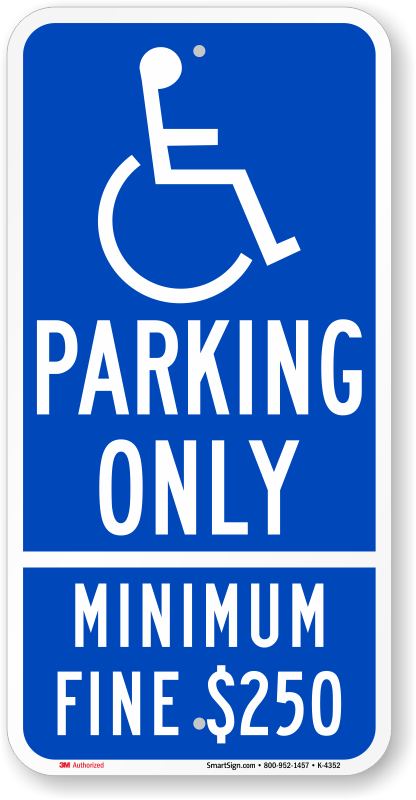The image depicts a rectangular handicapped parking sign, predominantly dark blue with a thin white border. At the top of the sign is a white drawing of a stick figure person sitting in a wheelchair, representing accessibility for individuals with disabilities. Below this symbol, the text "PARKING ONLY" is clearly printed in white capital letters, indicating that the space is reserved exclusively for handicapped parking.

A thin white line separates the top section from the text below. The sign sternly informs readers of a "MINIMUM FINE $250" for non-compliance, with the dollar amount prominently displayed. Further, detailed information is printed in red and black at the bottom of the sign within the white border. It includes the text "3M AUTHORIZED" in red, "SMARTSIGN.COM" in black, and a phone number "800-952-1457." Additionally, there's a black circle and the model number "K-4352," indicating the sign’s specific type or order number. The sign is also prepared with pre-drilled holes for easy mounting.